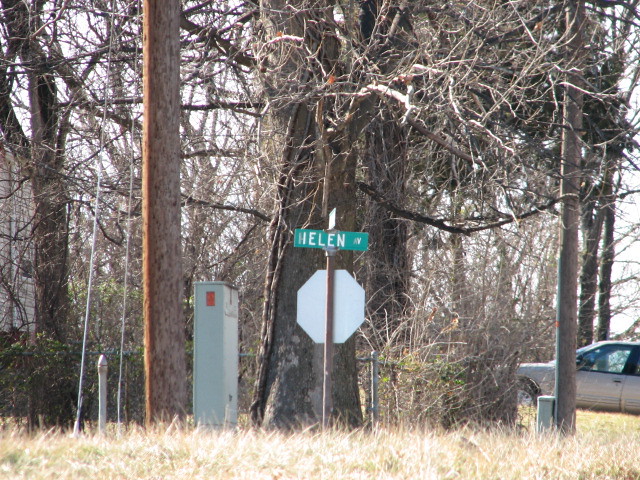A clear daytime outdoor scene depicts a suburban intersection dominated by a stop sign, viewed from behind. Above the stop sign, a street sign reads "Helen Avenue," and the image does not reveal the opposite side of the street. Adjacent to the stop sign is an electrical box positioned near an electrical pole, both of which are overshadowed by a large, leafless tree with sprawling branches. To the left, part of a beige house is visible, creating a backdrop of modest residential architecture. On the right side of the image, a driveway captures the attention where a four-door car, either white or light beige in color, is parked. Nearby, a second light pole stands, further characterizing the quiet, residential neighborhood setting.